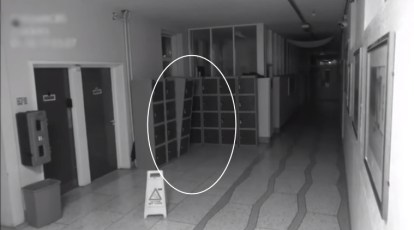The image, captured by a CCTV camera, shows a monochrome hallway scene with several distinct features. On the left side are two doors labeled for restrooms, one marked for ladies and the other for men. Adjacent to the doors is a device or box mounted on the wall, with a dustbin located directly beneath it. The hallway floor is lined with four irregular, scattered stripes and has a triangular hazard sign with a flat top. In the background, closed cabinets run along the wall, with one cabinet conspicuously tipping forward, circled by an oval highlight, indicating it as the focal point. Numerous picture frames adorn the right-hand side of the hallway, which extends into the distance. The overall perspective is landscape, about one and a half times wider than it is tall, reinforcing the sense of depth in this indoor setting.